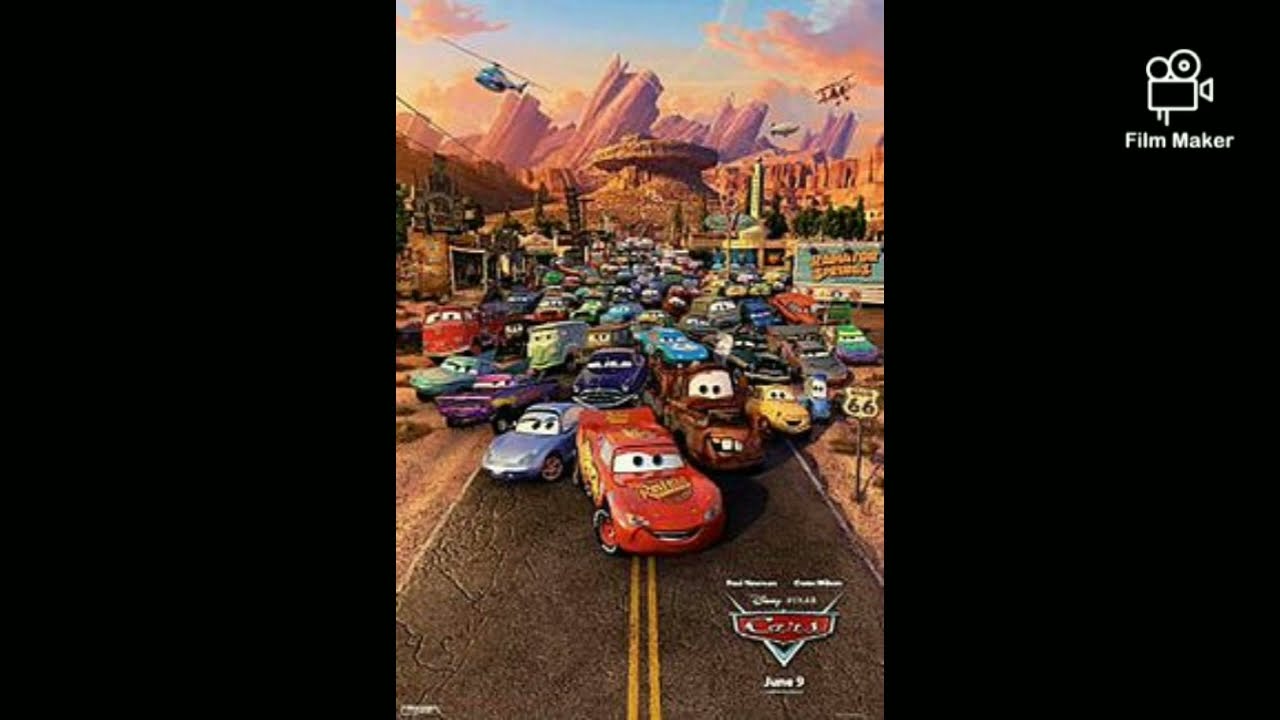The image is a detailed movie poster for the Disney Pixar film "Cars." It is in a wide rectangular format with the main poster in the center, surrounded by large black rectangles on either side. The poster showcases a variety of animated vehicles with expressive faces, all looking toward the camera, crowded together in the foreground. The primary character, Lightning McQueen, a bright red car, stands prominently at the front, accompanied by a multitude of other colorful cars, including a rusted tow truck, blue cars, and purple cars. They are positioned on a blacktop highway marked by yellow vertical stripes, set against a desert landscape featuring brown rocky mountains, cacti, and a prominent Route 66 sign. Above the scene in the sky, a blimp, an airplane, and helicopters are visible. The background also includes a light purple-brownish gray skyline, slightly toppled, beneath a bluish sky tinted with orange and pink clouds. The lower right corner of the poster features the emblem "Disney Pixar Cars" in silver, accompanied by the release date, June 9th. The upper right corner displays a white logo of a film camera with the word "Filmmaker."